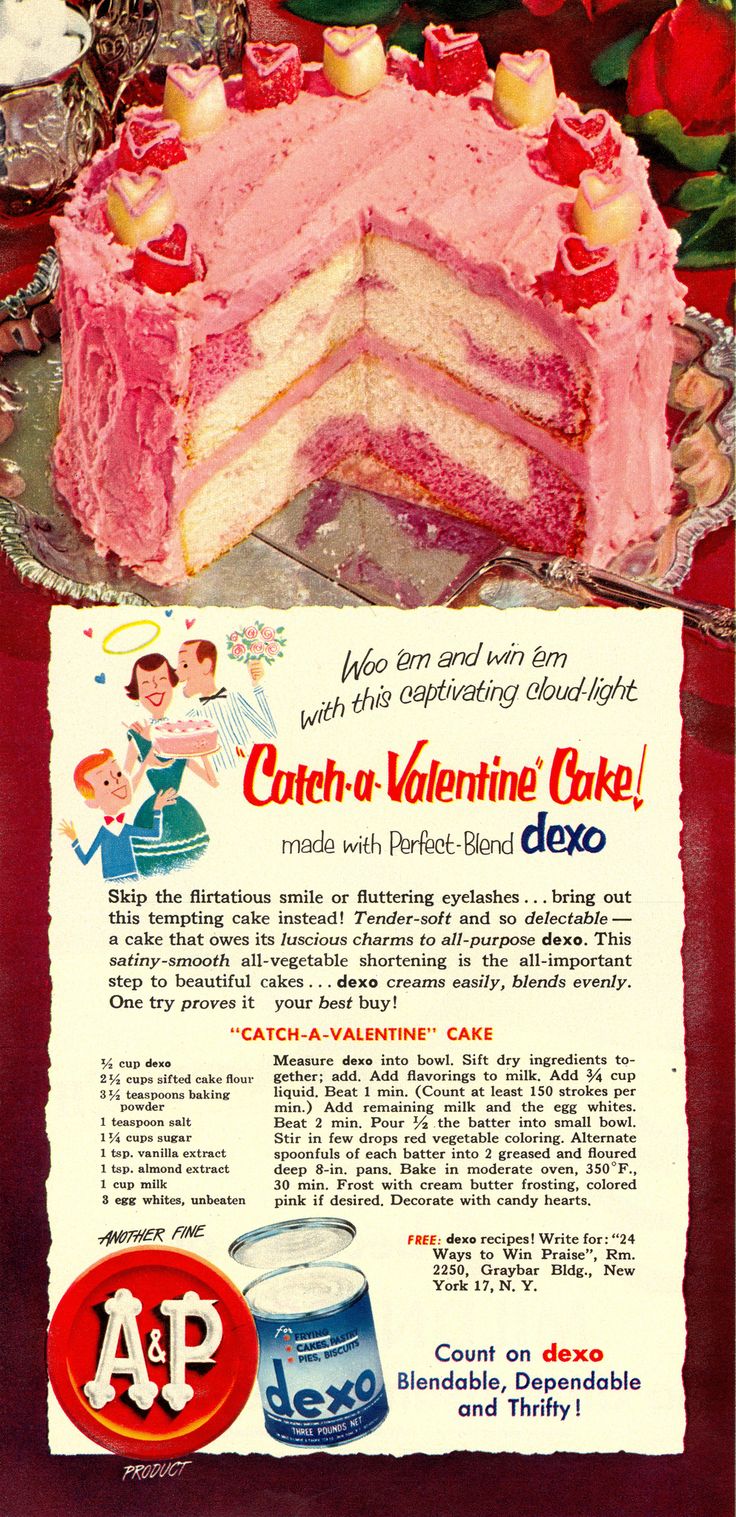This vintage advertisement, likely from the 1940s or 1950s based on the attire of the illustrated characters, features a two-layered, pink strawberry and vanilla cake with slices cut out to reveal its delicious interior. The cake, adorned with pink and white roses and heart-shaped candies, sits elegantly on a silver platter against a red backdrop. Above the cake, the text reads, "Woo them and win them with the captivating cloudlight, catch-a-Valentine cake made with the perfect blend Dexo." Below is a charming cartoon of a family: a woman holding the cake, a man offering flowers, and an eager little boy looking forward to a slice. The advertisement highlights Dexo, a blendable, dependable, and thrifty shortening, showcased in a blue can with its lid off, alongside a red circle that marks it as an A&P product. Tantalizingly, the bottom section provides the complete recipe, inviting readers to try their hands at this tempting Valentine treat.